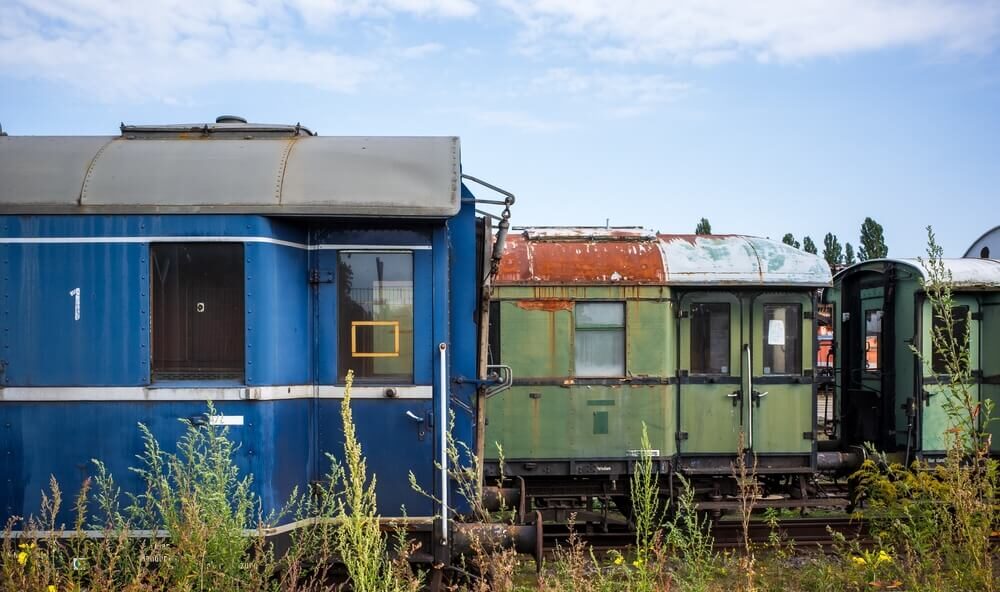The image depicts an outdoor railyard filled with disused and weathered train cars, surrounded by an overgrown landscape of tall green weeds. In the foreground to the left, there is a blue train car, which features two windows and has a gray roof showing signs of rust at the screw areas. This train car also has white stripes along its bottom, middle, and top sections. Behind it, to the right and in the middle distance, are two green train cars in much worse condition. These cars are heavily rusted, with the roofs covered in rust and one car even having double doors. The light blue sky above is mostly clear with a few white clouds, adding to the sense of abandonment. The overall scene conveys a sense of neglect and the passage of time, as none of the train cars appear to have been in use recently, and the tracks themselves are old and rusty.